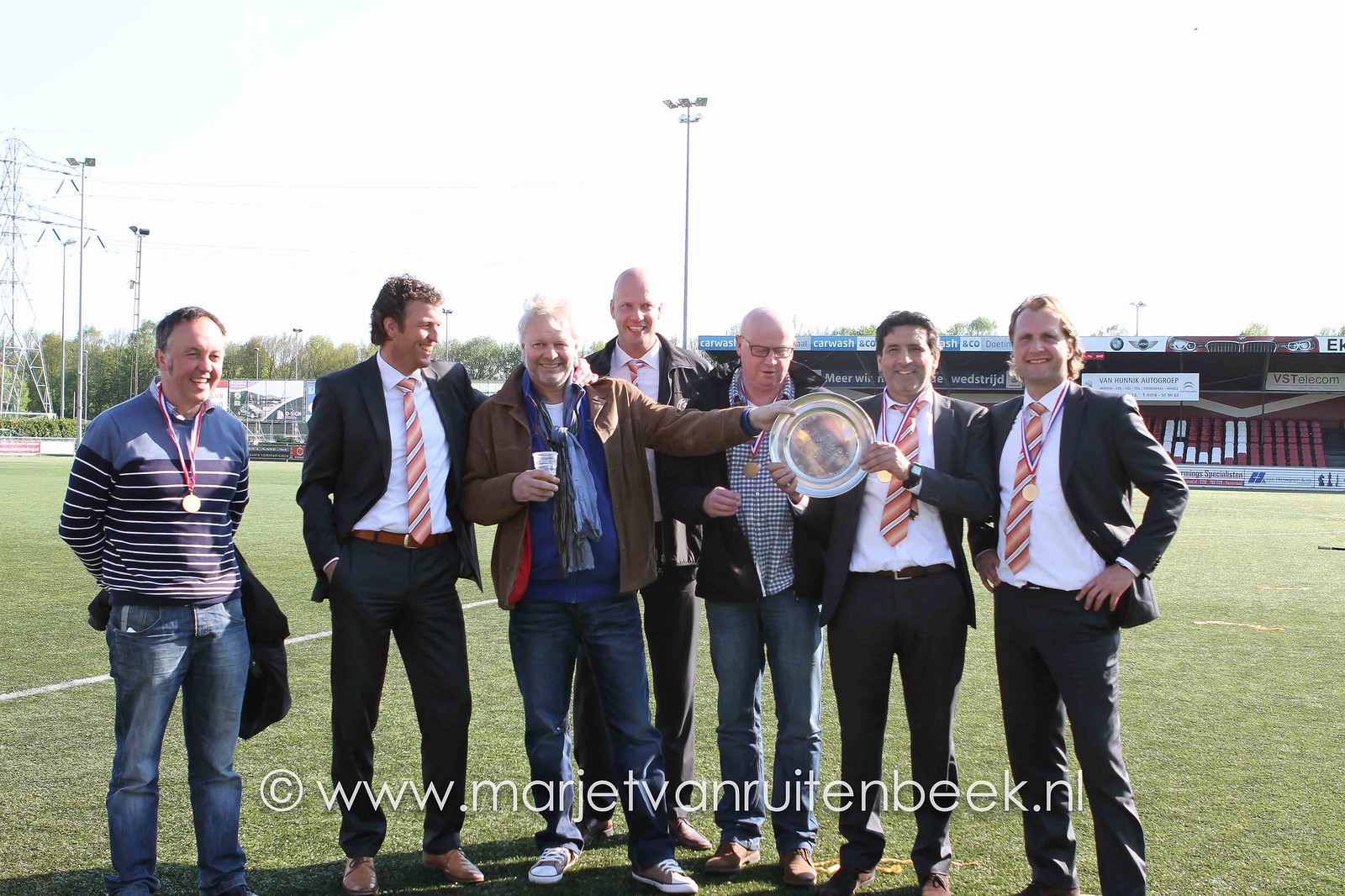In this image, set on a green, sunlit soccer field, eight athletic-looking white men, mostly in their 30s, gather for what appears to be an award ceremony. Most of them sport coordinated outfits—white shirts paired with orange-striped ties, brown jackets, and pants. Prominently featured are gold medals around their necks, indicating a recent athletic achievement or recognition event. The group includes two bald men and a mix of those with brunette and gray hair. Notably, one man on the far left diverges from the predominant attire, opting instead for a leather coat, blue shirt, and jeans, while another man, clean-shaven with curly hair, dons a full suit and tie. One individual, with a jubilant smile, holds a silver plate or trophy in his left hand and a glass in his right. The scene is vibrant and detailed, with background elements like stadium bleachers, light poles, and distant trees adding to the festive, yet relaxed post-ceremony atmosphere. A web address at the bottom hints at more information available online.